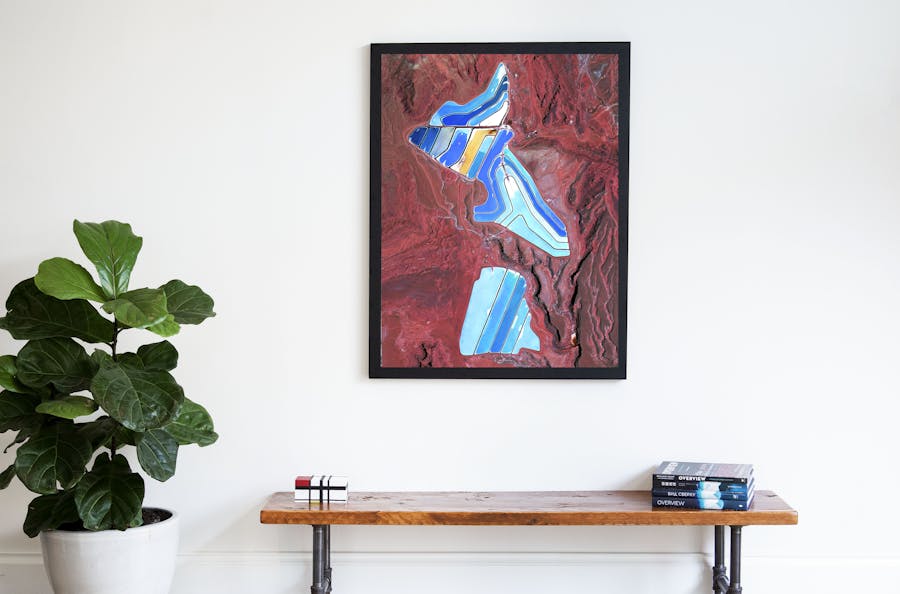The image portrays a serene waiting room or a stylish interior space, set against a stark white wall that appears greyish in the corners due to the lighting. Central to the composition is a painting in a black frame, featuring a purplish-red, abstract marble-like background interspersed with vivid squiggly lines in hues of light blue, dark blue, yellow, and white. The painting exudes a sense of refined modern art, potentially depicting a landscape or abstract scene with a satellite view resembling reddish mountainous formations, contrasted by segments of stained glass-like shapes. Below the painting is a wooden bench with steel legs, possibly a finished oak, doubling as a table. To its right, a neatly stacked pile of four books can be seen, and to the left is a curious object that may be another stack of books or an abstract white device with black stripes and a red mark. Flanking the setting to the left is a prominent green plant with broad, shiny leaves, housed in a white pot. The plant's lush foliage adds a natural, refreshing touch to the otherwise minimalistic yet tranquil space.